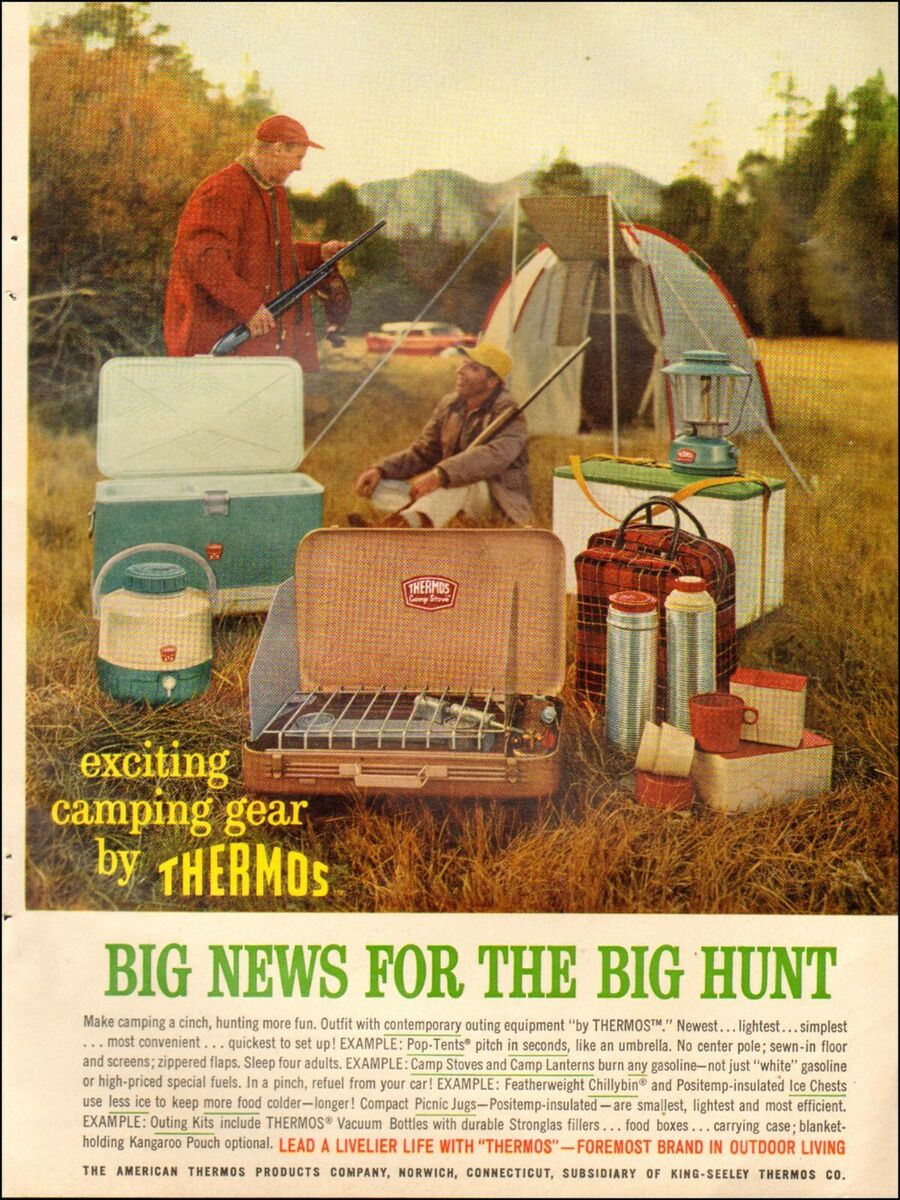In this vintage print advertisement for Thermos, set against a backdrop of an early 1960s woodland campsite, two white male hunters are featured. One stands clad in a red jacket and matching cap, gripping a shotgun in his right hand. The other, seated beside him, wears a brown jacket and yellow cap, with his rifle resting against his left shoulder. Surrounding them is an array of Thermos camping gear, including a water jug, cooler, camp stove, lantern, various thermoses, cups, and small containers. A tent is pitched nearby, and an early 60s car is partially visible in the background. The caption reads, "Big News for the Big Hunt," emphasizing the ad's appeal to hunters and campers. Detailed product descriptions are provided by the American Thermos Products Company, Norwick, Connecticut, a subsidiary of King-Select Thermos Co. The scene is realistic and meticulously staged, capturing the essence of a successful hunting trip with convenient and innovative Thermos equipment.